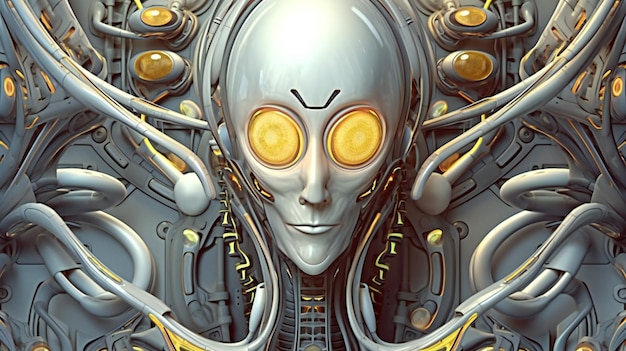This detailed digital artwork captures a sci-fi-themed robotic head centered in the image. The head features prominent, glowing bright yellow eyes that are disproportionately large compared to the rest of the face. Above the eyes, a V-shaped inlet cut adds a distinct, futuristic touch. The robot's face is defined by a well-sculpted nose, closed lips, and a thin jawline, culminating in a wide, light silver-colored head. Wrinkle-like details contribute to the face’s mechanical realism. Surrounding the head are numerous white tubes and cables accented with yellow, extending into the background filled with additional machinery. The entire composition exudes a metallic and glassy texture, consistent with a high-tech, sci-fi aesthetic often seen in H.R. Giger-inspired designs. This illustration appears to be a sophisticated computer-generated artwork, unaccompanied by any visible attribution or legible writing.